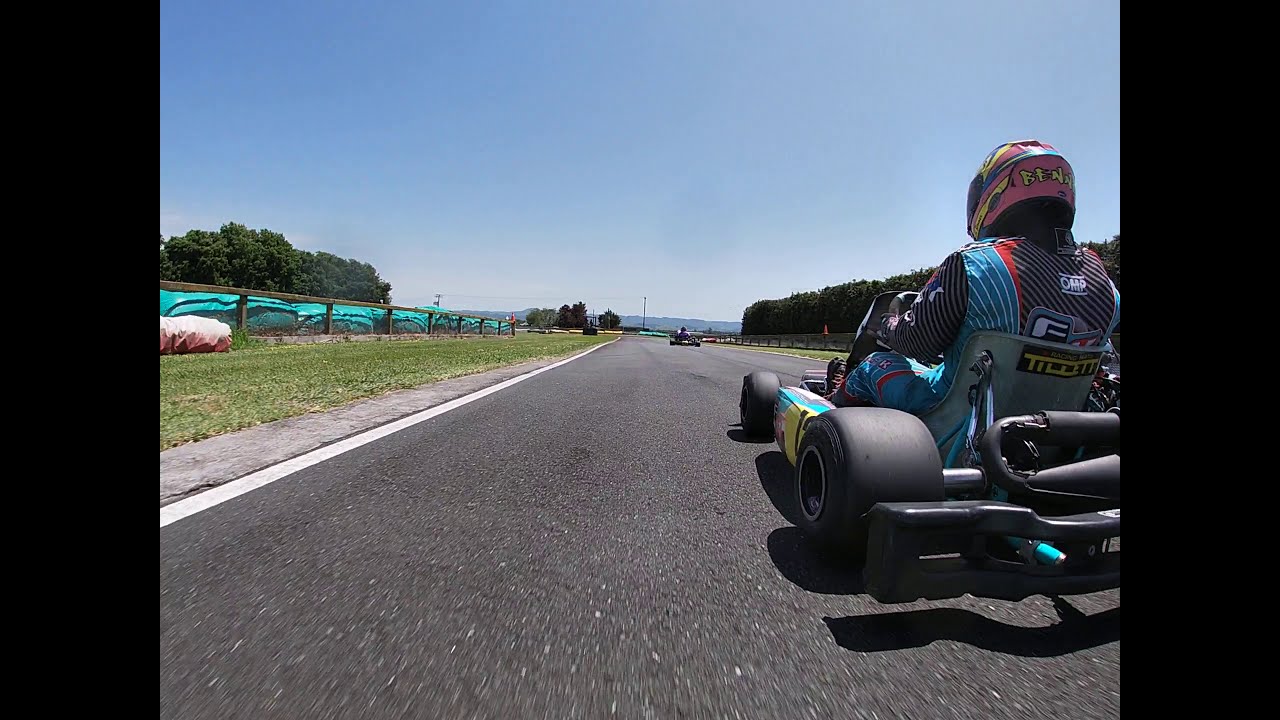In this vibrant photo of a go-kart race on a sunny day with a clear blue sky, we see the back of a driver navigating their go-kart close to the ground. The driver is equipped with a distinctive helmet adorned in pink, yellow, and blue. They wear a vivid outfit featuring red, blue, black, and white stripes. The scene is enriched with the go-kart's dynamic colors of gray, black, yellow, and green. Ahead on the asphalt track, more go-karts are visible, racing towards the horizon. The race course is wrapped by lush green trees on both sides, with railings and grass visible to the left of the track, creating a striking contrast against the brightness of the clear day.